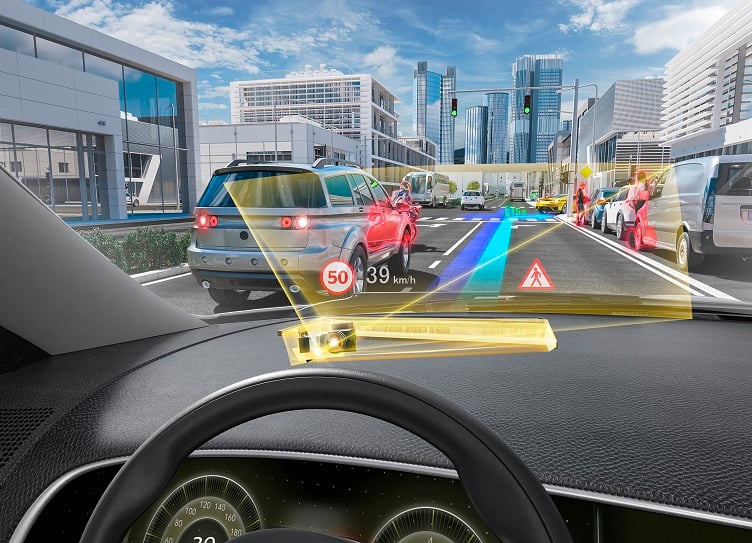This computer-generated image captures the view from the driver's seat of a car navigating through a busy city street. The top of the steering wheel and the dashboard are visible, showcasing a high-tech sensor system. This system includes a camera projecting data onto the dashboard with yellow beams highlighting various elements in the vicinity. The display provides critical information such as a "50" mark and a "39 kilometers per hour" speed indication, both pointing to different cars ahead. Additionally, a red hazard triangle with a pedestrian stick figure signals the presence of a person near the street, cautioning the driver. The scene outside shows a three-lane road with a bustling environment: cars traveling and parked, a pedestrian, a distant bus, and towering skyscrapers. The overall image illustrates the advanced capabilities of the car's sensor to measure distances, detect pedestrians, and provide real-time traffic updates, emphasizing the integration of safety features in a futuristic urban setting.